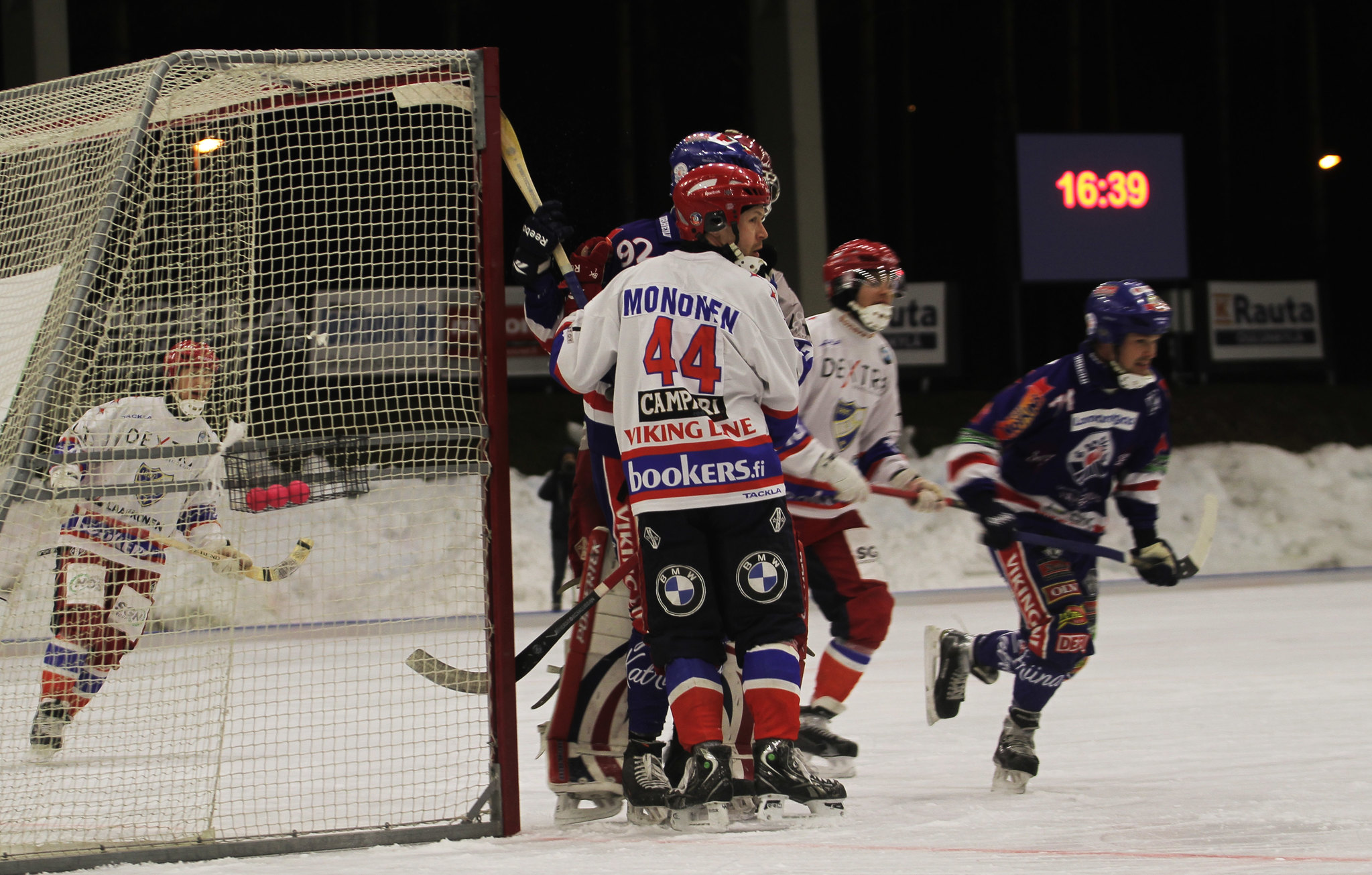In the image, a group of five or six men are playing hockey on an outdoor rink, likely at nighttime. They are fully equipped in hockey gear, including helmets, skates with black boots and white laces, and are holding hockey sticks. The scene is framed by a white goal on the left side, viewed from the side, while the top right corner features a digital clock with bright orange numbers displaying "16:39." The players are divided into two teams: one team with red helmets, white jerseys, and dark pants, and the other team with blue helmets and blue jerseys. In the background, various advertisements for "RAUTA" are visible against a white backdrop. Snow, mixed with some dirt, is piled on the outskirts of the ice rink. The setting is quite dark, with a faintly illuminated sign in the background marking the time, adding to the nighttime ambiance.